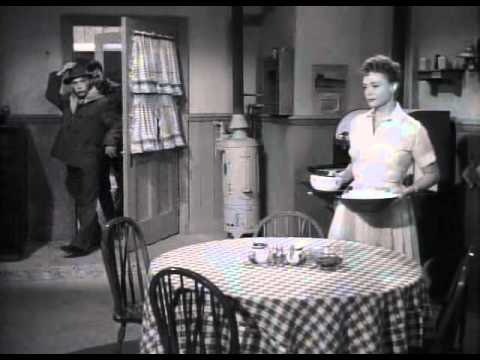The image is a black and white still from what appears to be a 1950s TV show or movie. It depicts an indoor scene in a house where a woman, dressed in a short-sleeved, collared white dress, stands by a kitchen table covered with a gingham-checked tablecloth. She holds two dishes in her hands and exhibits a thoughtful expression, accentuated by her short curly hair. Surrounding the table are four wooden chairs. In the background, a door with window curtains is slightly ajar. Two men are entering through the door; the man in the foreground is in the process of removing his hat with his right hand and is dressed in a coat, pants, and black shoes. The second man, partially obscured, is also wearing a coat and hat. The scene suggests they might be arriving for dinner.